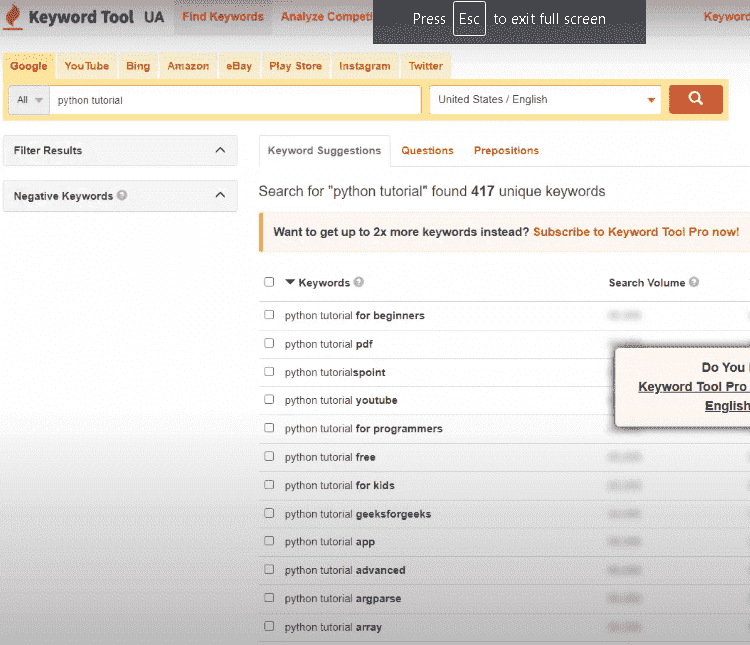This image appears to be a screenshot from a website with a white background. At the top left corner, various tabs are visible. The first tab, labeled 'Keyword Tool' in black text, signifies the name of the website. To its right are two tabs, one in orange text reading 'Find Keywords' and another in black text likely saying 'Analyze Competition'.

Adjacent to these tabs is a semi-transparent gray box with white text, stating, "Press Escape to exit full screen". Below the 'Keyword Tool' tab, a row of yellow tabs is displayed, each corresponding to different search platforms including 'Google', 'YouTube', 'Bing', 'Amazon', 'eBay', 'Play Store', 'Instagram', and 'Twitter'.

Beneath this row, two white boxes are displayed. The left box contains the text 'Python Tutorial' in black, while the right box displays 'United States / English'. Directly below this, there are three more tabs, the first of which, in gray text, is labeled 'Keyword Suggestions'. To its right, orange text labels the other two tabs as 'Questions' and 'Prepositions'.

Further down, gray text indicates search results with the message, "Search for Python Tutorials, found 417 Unique Keywords". Below this statement, a list of keywords is presented in separate rows. The keywords listed include:
1. Python Tutorial for Beginners
2. Python Tutorial PDF
3. Python Tutorials Point
4. Python Tutorial YouTube
5. Python Tutorial for Programmers
6. Python Tutorial Free
7. Python Tutorial for Kids
8. Python Tutorial Geeks for Geeks
9. Python Tutorial App
10. Python Tutorial Advanced
11. Python Tutorial ArgParse
12. Python Tutorial Array

This detailed view underscores the analytical focus of the website, aimed at providing comprehensive keyword research and analysis tools primarily for SEO and content creators.